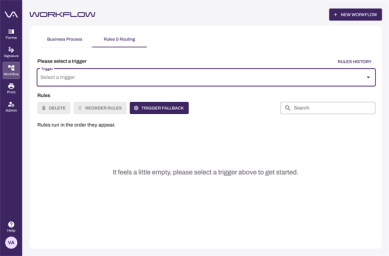This image, sourced from a web page, showcases a user interface focused on workflow management. Dominating the left side is a broad purple rectangle stretching vertically from top to bottom, clearly labeled "Workflow" in bold, purple typography at the top. Within this purple section, there's a clickable box labeled "New Workflow" also in purple.

The overall background is a faint gray, providing a subtle contrast to the upper section's white backdrop. The interface is accented by various purple elements for visual continuity. In the upper part of the interface, a noticeable feature is the "Trigger Fallback" text.

Central to the white area, towards the lower middle, is an empty section highlighted by the message, "It feels a little empty, please select a trigger above to get started." This empty section features a prominent purple, elongated rectangle with the directive "Please select a trigger." Inside this rectangle, there is a drop-down menu labeled "Select a trigger," inviting user interaction to proceed with the workflow setup.